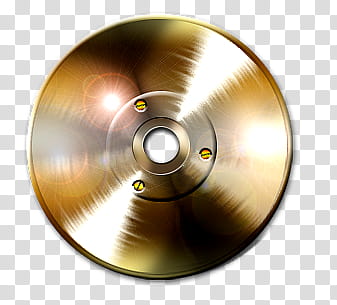The image features a dark gold disc with a grooved surface, closely resembling an old-fashioned record. This disc is centered on a grey-and-white checkered background, which is visible through a hole in the very middle of the disc, akin to that of a vinyl record. Surrounding this central hole is a small, solid gold ring, followed by another ring within which three flathead screws are symmetrically set. Light reflections on the disc enhance its metallic sheen, emphasizing the intricate detailing of the grooves and the overall structure of the disc.